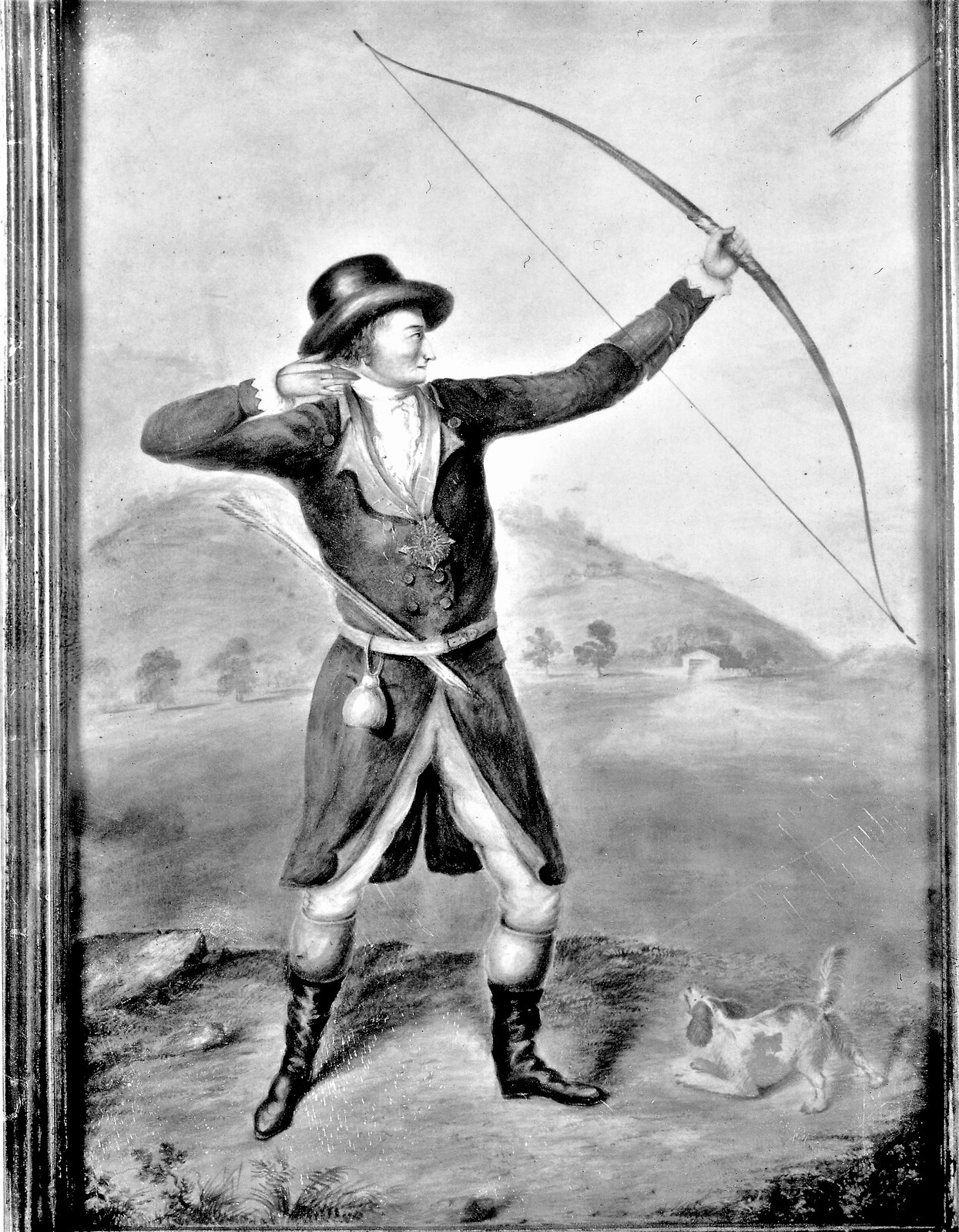This black-and-white image, seemingly aged and worn with tattered edges, appears to be a photograph or a painting from an old book. It captures a man, dressed in 1700s or 1800s colonial attire, standing on a small grassy hill with a backdrop of a grayscale sky. He wears a black top hat, a long black coat down to his knees with lapels shaded in gray, and a frilled white shirt. His outfit is completed by puffy white leggings and tall boots with white socks peeking out. Around his waist, a belt holds a pouch filled with arrows. The man holds a bow in his left hand, and an arrow he has just released is visible in the upper right corner of the image. At his feet, a small two-toned, white and gray dog is in a playful stance, down on its front paws with its back paws and butt up in the air, possibly barking or watching something. Additionally, a faint picture frame can be seen on the left side of the image, adding to its historical feel.